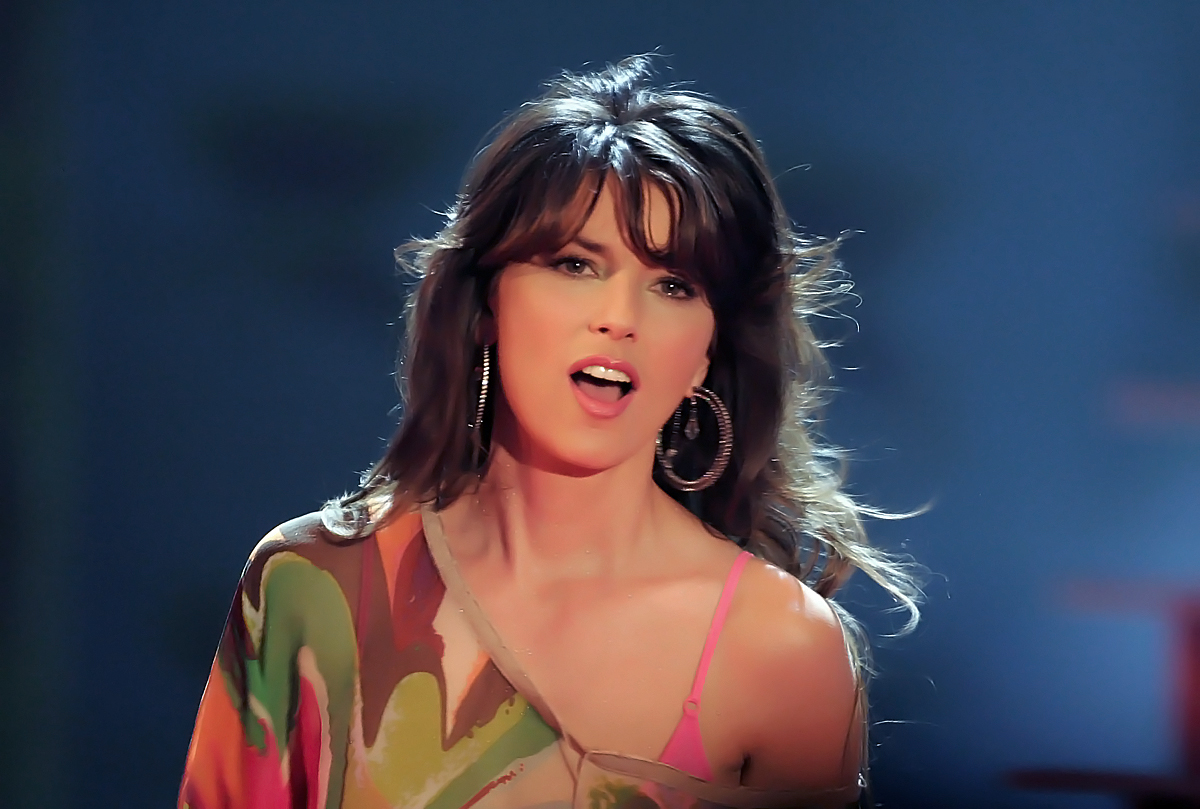This horizontally aligned rectangular image features a woman, possibly an actress or singer, centered in the frame from about the chest up. The background is a blurry gradient of blue, with darker shades predominantly on the left transitioning to lighter shades towards the right. The woman has a captivating, intense gaze directed at the viewer with her mouth open, suggesting she is in the midst of singing. Her brown eyes are accentuated with pink lipstick, revealing her top row of teeth.

She sports long, wavy brown hair with bangs, cascading down her back and over one shoulder. She is adorned with large silver hoop earrings that add a touch of elegance to her look. Her outfit consists of a patterned blouse draped over her right shoulder, blending hues of green, brown, orange, and beige, resembling brushstrokes. On her left shoulder, a pink spaghetti strap is visible, hinting at a tank top or bra beneath the blouse. This ensemble, combined with the blurred yet vibrant background, places her as the striking focal point of this image.